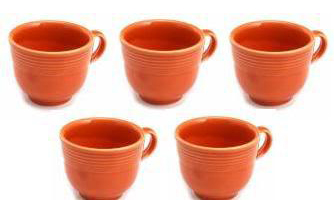This image showcases five identical coffee mugs, all meticulously arranged to resemble mirror reflections of each other, giving the impression that they might have been digitally multiplied. Each mug has a small, looped handle and is decorated with subtle circular ridges around the top inch, adding a slight decorative flair to their otherwise simple design. The mugs have a terracotta-like, reddish-orange exterior and a slightly darker interior, suggesting a pottery make, although they might also be made of plastic. Positioned in a uniform fashion—three on top with two beneath—and set against a plain white background, these small-sized mugs, perfect for a cup of tea or coffee, emphasize symmetry and simplicity while inviting a sense of cozy functionality.